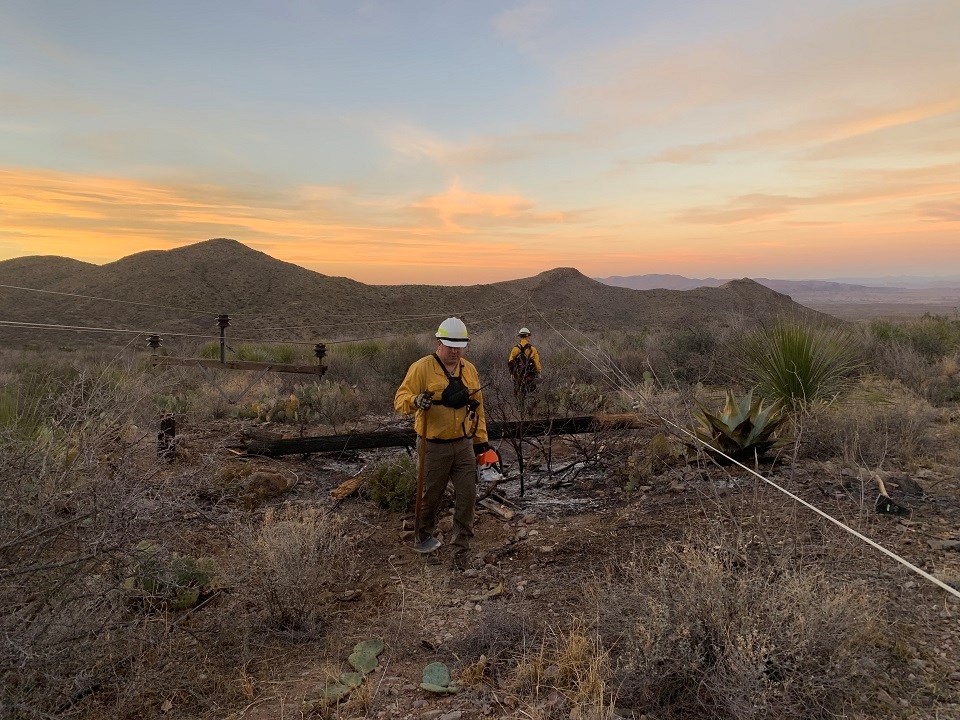In this photograph, two workmen can be seen in a desolate, desert-like landscape. The foreground features a man in brown pants, a yellow shirt, white hard hat, and gloves, holding what appears to be a shovel as he walks towards the camera. A second man, also dressed similarly with a hard hat and equipped with a backpack, stands further back with his back facing the photographer. In the center of the image, a power pole lies horizontally on the barren ground, charred and broken, with its detached crossbar and lines still visible on the desert floor.

The background offers gently undulating dirt hills with no greenery, progressing into distant, higher hills or mountains. The sky above adds drama with streaking clouds illuminated by the colors of dusk: an amber glow on the horizon transitioning to an orangey-pink, and finally, a darkening blue expanse. The dry landscape features minimal vegetation, including sparse cacti and potentially an aloe plant. This image captures a moment of repair or inspection in the isolating vastness of a post-disaster desert setting.